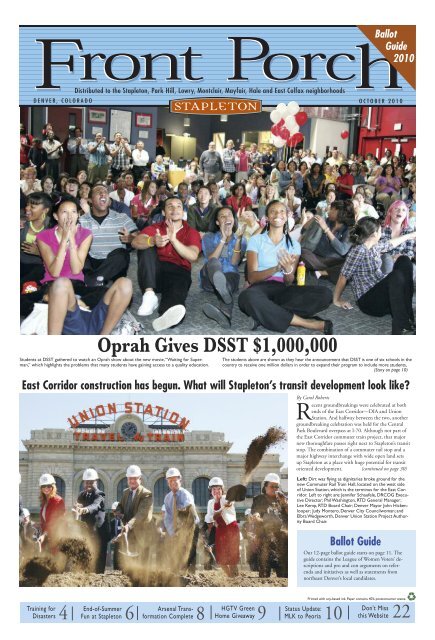The image depicts the front page of the *Front Porch* magazine, dated October 2016. The magazine features a blue background with black and yellow writing and is distributed in the Stapleton, Park Hill, Lowry, East Collins, and other Denver neighborhoods. In the top corner, there is a label reading "Ballot Guide 2010." The main image shows a diverse crowd of young people sitting on the ground, with some clapping and cheering, underscored by the headline "Oprah Gives DSST $1 Million." Below this, another headline reads, "East Corridor Construction Has Begun: What Will Stapleton's Transit Development Look Like?" accompanied by a photograph of people in business attire and white construction hats, shoveling dirt at Union Station, signifying the start of the construction. Additional information is contained in a small blue box labeled "ballot guide," though the text is too small to be legible.